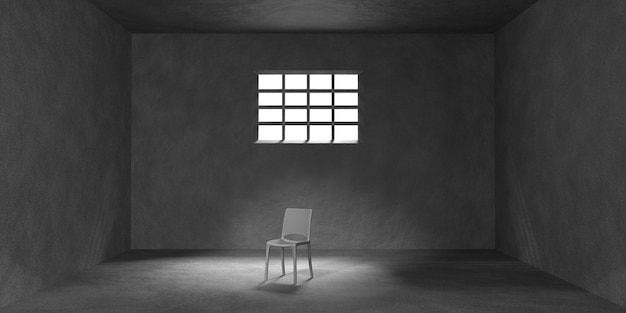This detailed artist's drawing, rendered in a grayscale palette, portrays a minimalist and somewhat melancholic room. The room's walls are slightly skewed, creating an optical illusion that mimics the effect of a convex lens or panoramic view. Central to the artwork is a solitary, simple plastic chair placed prominently in the middle of the room, bathed in soft, glowing light streaming through a multi-pane barred window on the gray rear wall. The window, divided into a grid by three vertical and three horizontal bars, casts shadows and adds to the austere ambiance, lending the scene an almost prison-like feel. The light also reflects faintly on the ceiling and chair, amplifying the stark contrasts and shadows that dominate the room. The overall setting, devoid of any people, evokes a sense of emptiness and solitude, capturing the viewer's attention through its subtle details and somber tone.